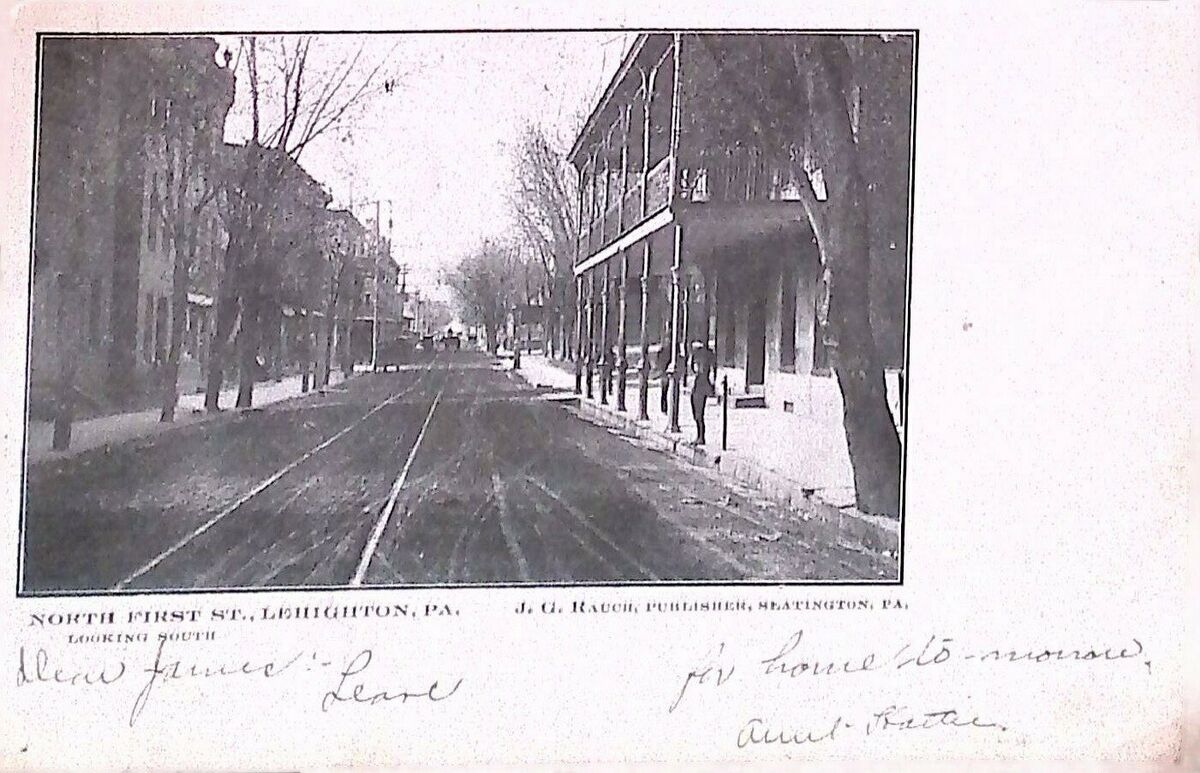The image is an old, black and white postcard featuring a scratched and grainy photograph of North First Street in Lehighton, Pennsylvania, as indicated by the cursive writing on the reverse. The scene is looking south and showcases a mix of architectural styles. On the right side of the street, there's a two-story building with a balcony and railing reminiscent of New Orleans' Bourbon Street architecture. On the left, there are more standard buildings akin to those found in New York or Chicago. The street itself includes a rail track, possibly for a trolley, and posts along the sidewalk for hitching horses, reflecting an older time period. Leafless trees are present on both sides of the street. The photograph is accompanied by several written details including "North First Street, Lehighton, PA," "Looking South," and the photographer's name, J.G. Rauch. Below these, there are three signatures, including a Reverend, an Aunt, and a Drew. The back of the postcard is light pink, adding a subtle touch to its vintage charm.